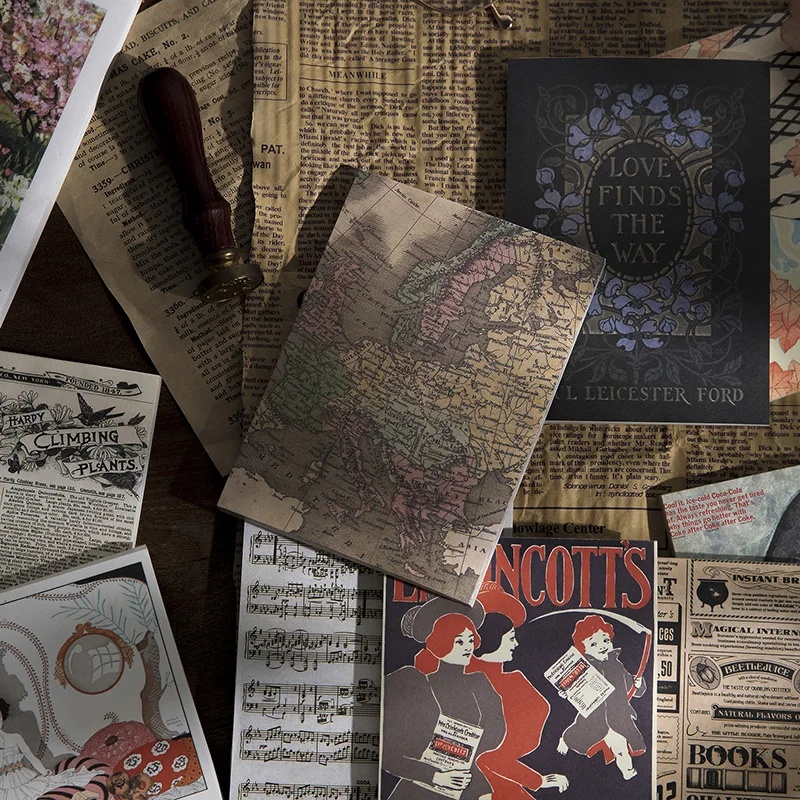The photograph, taken from above, showcases an array of vintage documents and items scattered irregularly across a table. At the center lies a distinctive map with bolded sections, providing a focal point. Surrounding the map are several timeworn newspapers and excerpts dotted with yellowing edges, hinting at their age. Notably, there is a book titled "Love Finds the Way" by L. Leicester Ford. Another book surfaces, displaying two women and a child on its cover, with the partial title "Indicots," and a third book featuring a world map. Among the papers are advertisements, including one promoting "Hardy Climbing Plants," and a sheet of music. An embossing tool with a brown handle and gold top is also prominently placed on the desk. Additionally, there are visual elements: a picture of flowers in the top left corner, an old photograph depicting a tree, an orb, and a woman in a dress. Furthermore, there is a wax seal stamp lying on the table, enhancing the vintage ambiance of the scene.